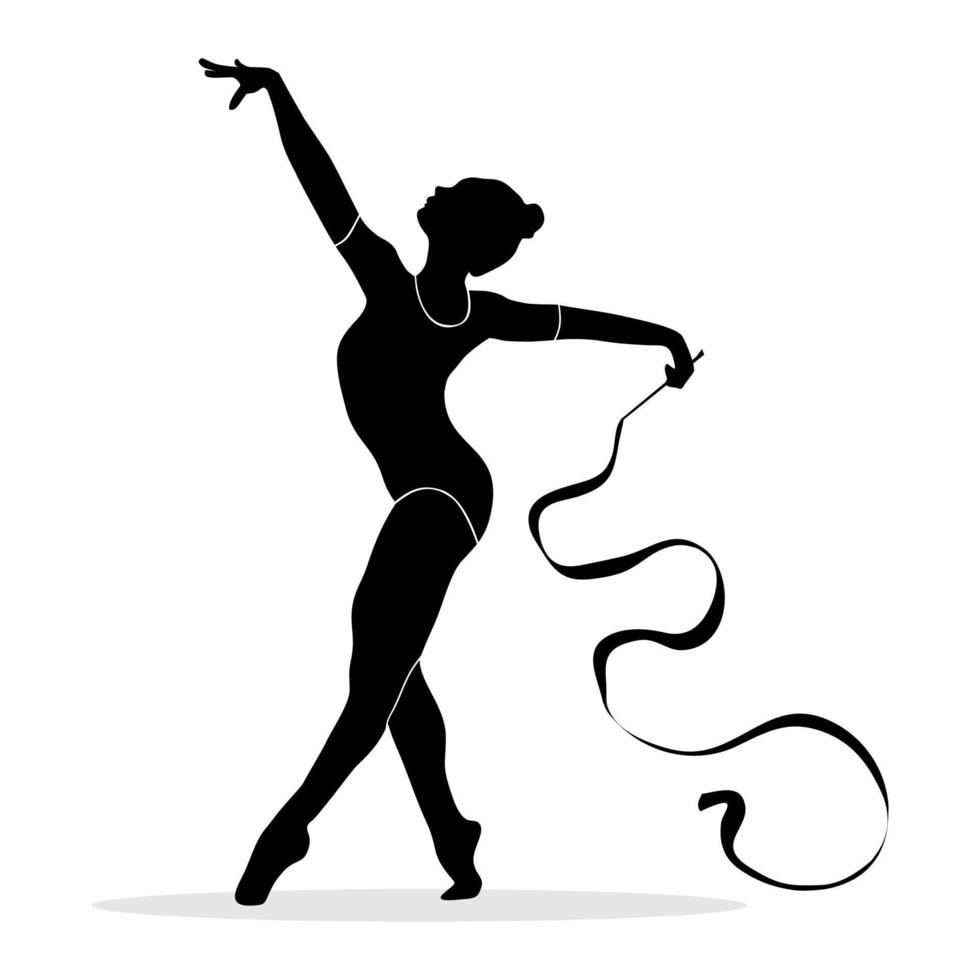The image is a black-and-white graphic featuring a central, vector-style illustration of a young woman or ballerina, holding a ribbon streamer in her right hand. The dancer's pose is dynamic; her left hand extends upwards at a 45-degree angle with fingers splayed, while her arched back and upward-tilted head convey a sense of grace and motion. Her right leg is bent, and she stands on the ball of her right foot, appearing to be mid-dance or striking a gymnastic pose. The background is entirely white, emphasizing the elegance and fluidity of the dancer's form against the stark, uncluttered space.